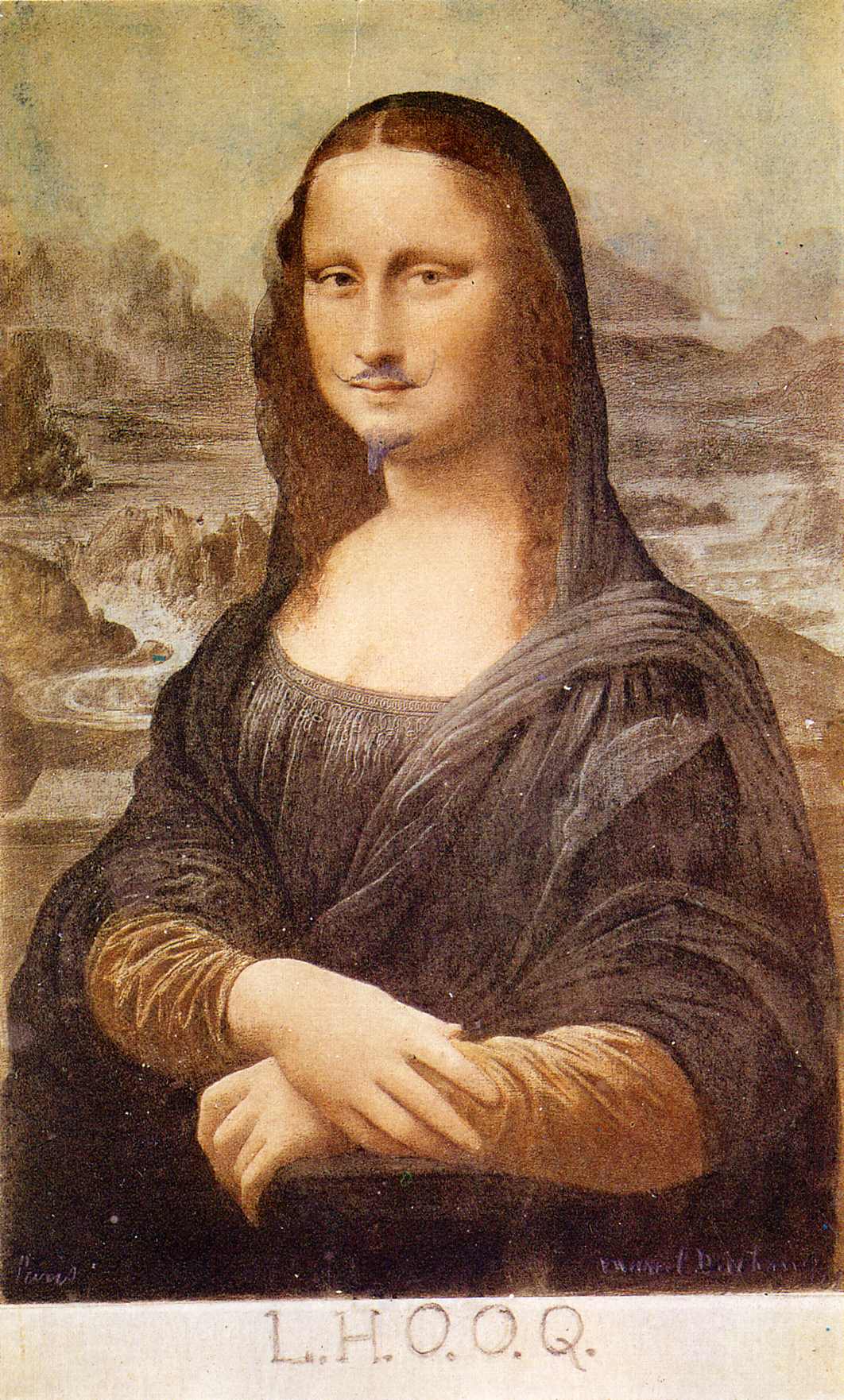In the rectangular image, approximately twice as tall as it is wide, we see a playful rendition of the classic Mona Lisa. The painting retains its iconic elements: the centered figure of the Mona Lisa with her enigmatic expression, shoulder-length dark brown hair, and her hands gently crossed in front of her, dressed in a dark garment revealing her upper chest and neck area. However, a notable deviation from Da Vinci's original is the addition of a handlebar mustache and a long goatee, both in a dark gray hue, giving it a whimsical twist. 

The backdrop maintains the traditional landscape, featuring an open field with bushes and plant life that transitions into what appears to be a mountainous horizon with gray and white shapes, under a yellowish-gray sky. 

At the bottom of the image is a white band, almost forming a border, centered with dark gray text reading "L.H.O.O.Q." The color palette follows the classic tones of the original painting, with shades of gold, gray, peach for her skin, and various browns in the background, layered to enhance the blend of timeless artistry and humorous alteration.